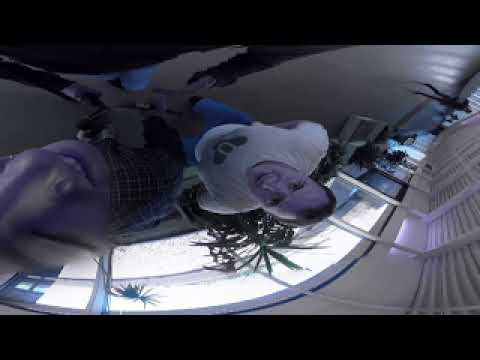The fisheye lens image appears to be taken inside a bright, white-walled space, possibly a house, event center, or office building lobby. The image is somewhat upside down and distorted, showing three people. The woman closest to the camera, wearing a plaid shirt, has a warped head possibly due to camera movement, and is smiling with partial teeth visible. To her right is a man in a white t-shirt and blue jeans, his face blurred but looking up at the camera. Slightly off-camera is another person wearing a black long-sleeve shirt and blue jeans. Natural light streams in from numerous windows, reflected on the glossy, light-colored flooring. Behind the group is a potted plant, possibly a palm tree, and a corridor with a white ceiling, contributing to the bright and airy feel of the space.